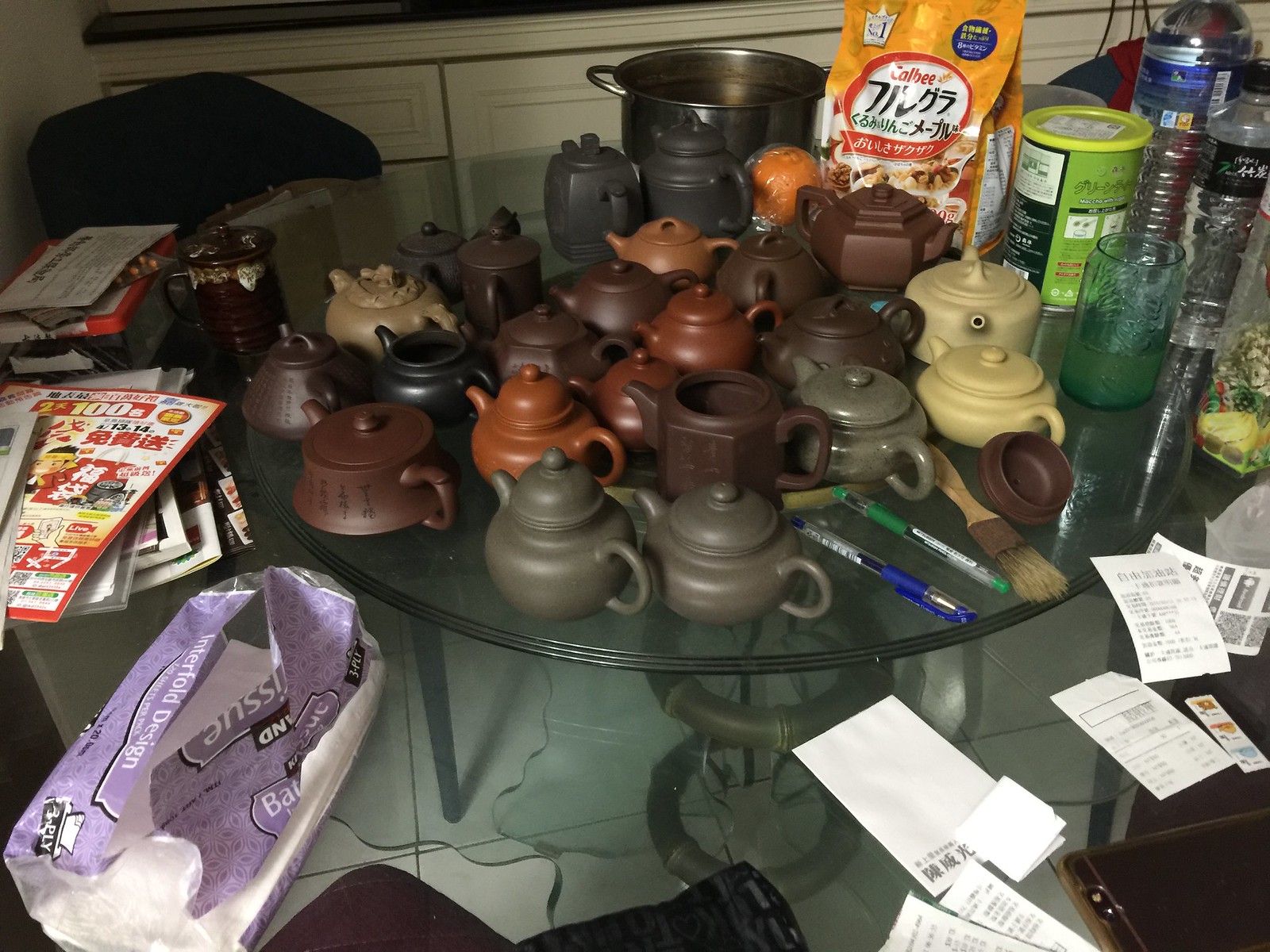The image depicts an array of small clay Chinese teapots spread across the surface of a round glass table with metal legs. The teapots, designed with handles, spouts, and covered tops, exhibit a variety of shapes including flat circular, spherical, cone-shaped, cubicle, and hexagonal forms. They come in shades of light to dark brown, olive green, orange, cream, and gray, with some featuring Chinese text either engraved or inscribed in black ink. The table is quite cluttered and includes numerous other items: on the right side, a pile of white receipts; on the left, a napkin with a pink plastic cover; and further left, some magazines with reddish and white covers. In the background, there's a silver cooking pot, clear plastic water bottles, and a yellow coffee packet with a red circle. Additionally, the table holds various bags and containers filled with food, some with Japanese writing.